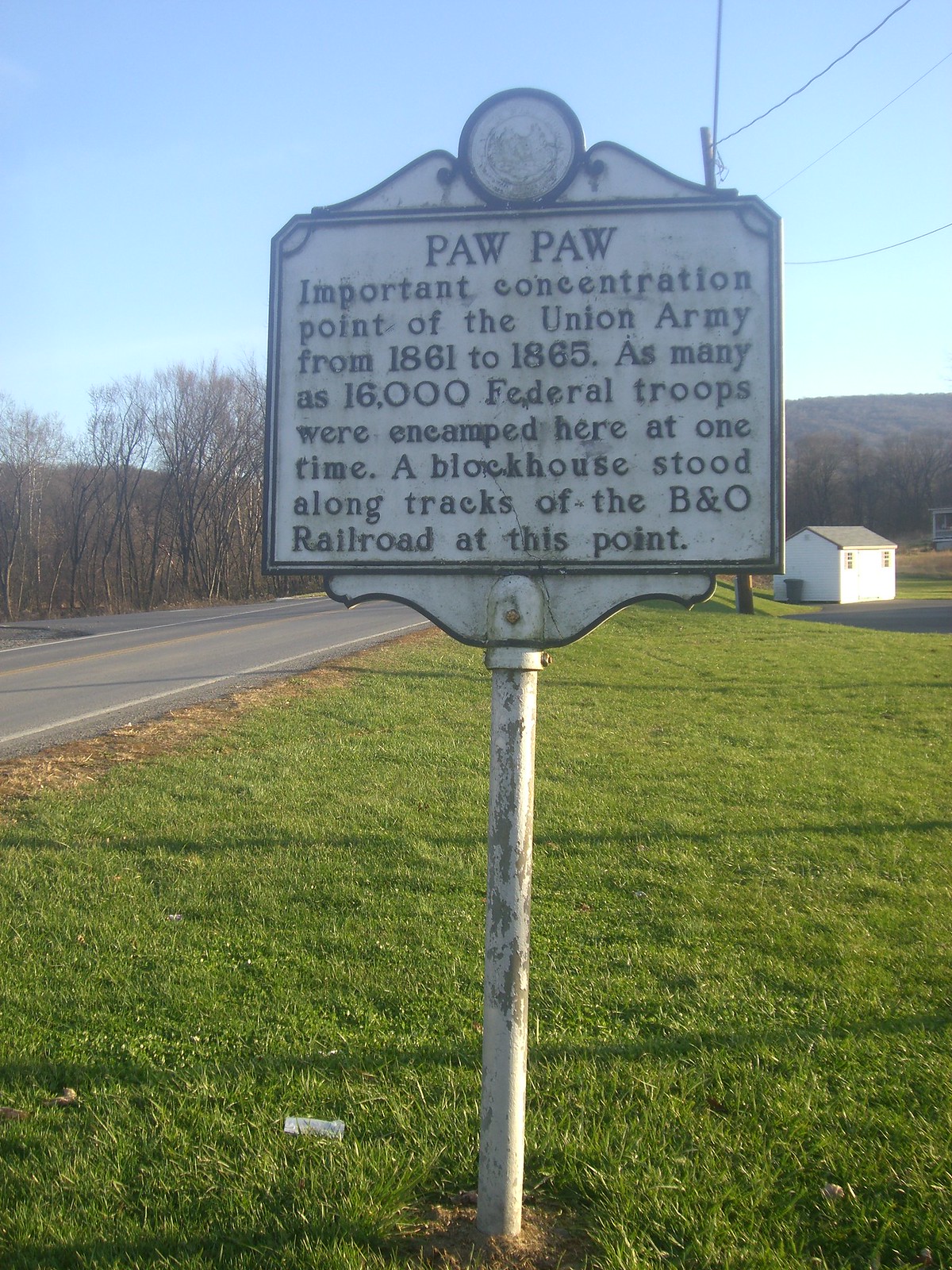The image depicts a historic marker in the center of a grassy field, flanked by a single-lane asphalt road to the left. The white rectangular placard is mounted on a metal pole, also painted white, and is noticeably deteriorated with rust and paint chipping away. The text on the marker reads: "Paw Paw, important concentration point of the Union Army from 1861 to 1865. As many as 16,000 federal troops were encamped here at one time. A blockhouse stood along the tracks of the B&O Railroad at this point." The backdrop includes a small white house with a gray roof to the right, distant trees, mountains, and power lines against a light blue sky, indicating a sunny outdoor setting.